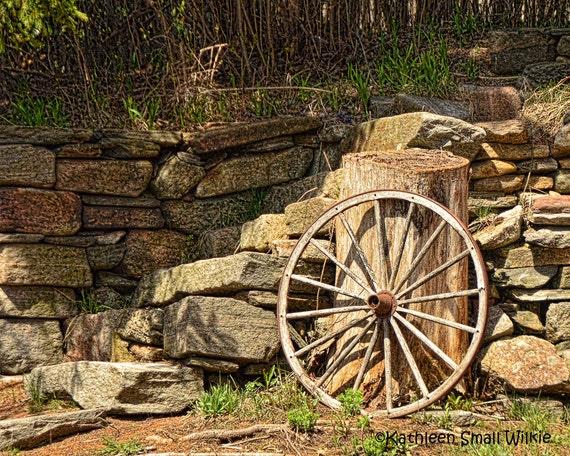The viewer is presented with a serene countryside scene, standing on a meandering path adjacent to a roughly constructed dry stone wall. The wall, composed of uncemented, weathered stones, exudes rustic charm. Centered in the image are a series of stone steps that ascend to an upper level, culminating in a lush expanse of grass and varied vegetation that crowns the background. In the immediate foreground, a sizable tree stump, nearly reaching the height of the wall, catches the eye. Leaning casually against the stump is an old wooden wagon wheel, complete with an iron tire and hub, adding to the bucolic atmosphere. Bathed in warm sunlight, the entire scene radiates a tranquil, rural beauty that is both inviting and picturesque.